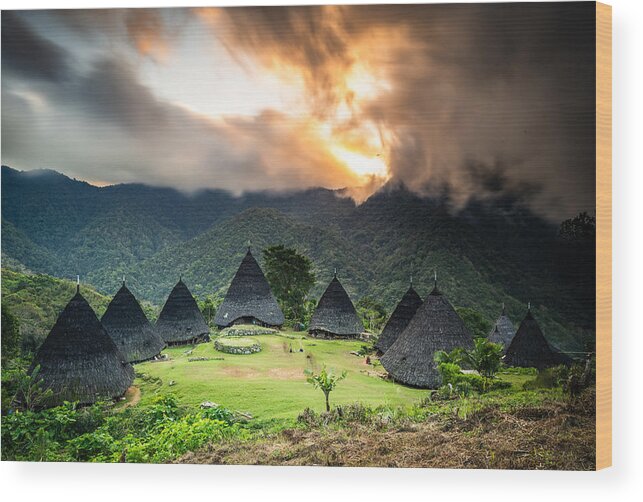This photograph captures an outdoor scene featuring a tribal village composed of nine large, conical huts arranged in a circular formation on a flat, grassy knoll. The huts appear to be constructed from natural, plant-based materials, likely thatched palm leaves, which give them a dark, greyish-black hue. Each structure is remarkably tall, possibly reaching up to 2 or 3 stories in height, and some have distinctive spikes or antennas protruding from the top.

The village is situated in a clearing on a hillside, with rough, rocky terrain in the foreground. Surrounding this clearing are rolling hills that transition into tree-covered mountains. The mountains, densely packed with green trees, create a striking backdrop and appear to be part of a larger mountain range. At the peaks, clouds gather, appearing foggy and in motion, partially illuminated by the setting sun. The sky is a canvas of dark grey, light grey, orange, and yellow hues, contributing to a dramatic and somewhat serene ambiance.

Adding to the complexity of the landscape, there are several tall, unidentified trees and palm-like trees interspersed among the huts. Directly in front of the village, there is a structure made of stone, circular in shape. The overall scene is rich in natural beauty, combining elements of rugged terrain, lush vegetation, and traditional architecture under a dynamic, colorful sky.